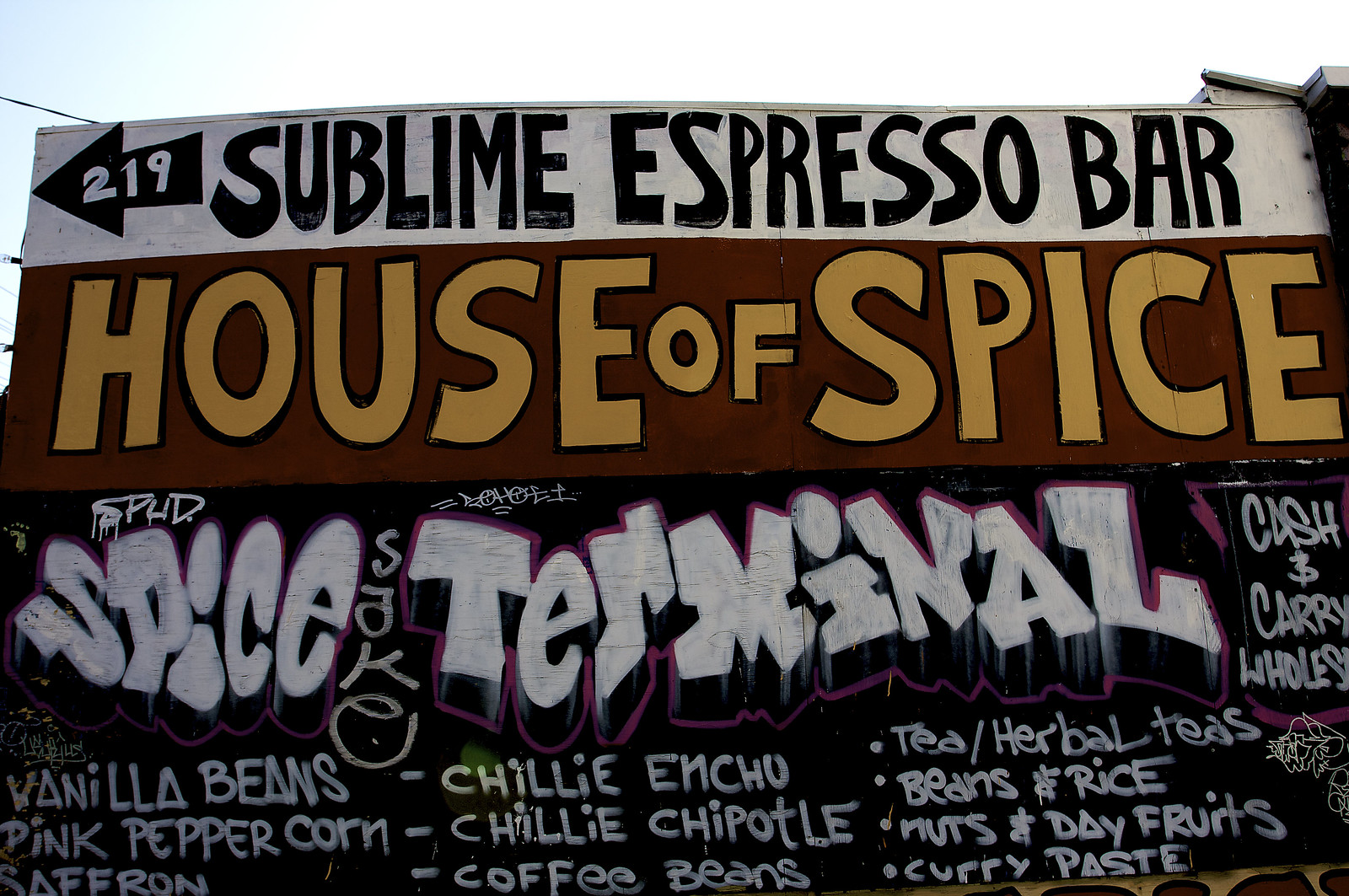The image features a photograph of a handwritten advertising menu board for the 219 Sublime Espresso Bar and the House of Spice. The sign is prominently displayed outdoor, perhaps in a bustling downtown district or near a beach lined with coffee bars and specialty shops, suggesting a vibrant, casual atmosphere. The sign itself is primarily black with white lettering, complemented by a red stripe with red and yellow lettering near the top, and a white stripe with black lettering at the very top.

The text is centered across the board, with "219" and an arrow pointing to the Sublime Espresso Bar and the House of Spice. The menu details various offerings in an array of white slightly uneven, handwritten text, perhaps chalk, which suggests it might be updated regularly. Listed items include vanilla beans, pink peppercorn, saffron, chili varieties (ancho and chipotle), coffee beans, tea, herbal teas, beans and rice, nuts, dried fruits, and curry paste. It also mentions "sake," "cash and carry wholesale," and "spice terminal," hinting at a diverse inventory aimed at both retail and wholesale customers. Some parts of the text might be hard to read due to the handwritten nature, adding a rustic, yet homey charm to the establishment's presentation.